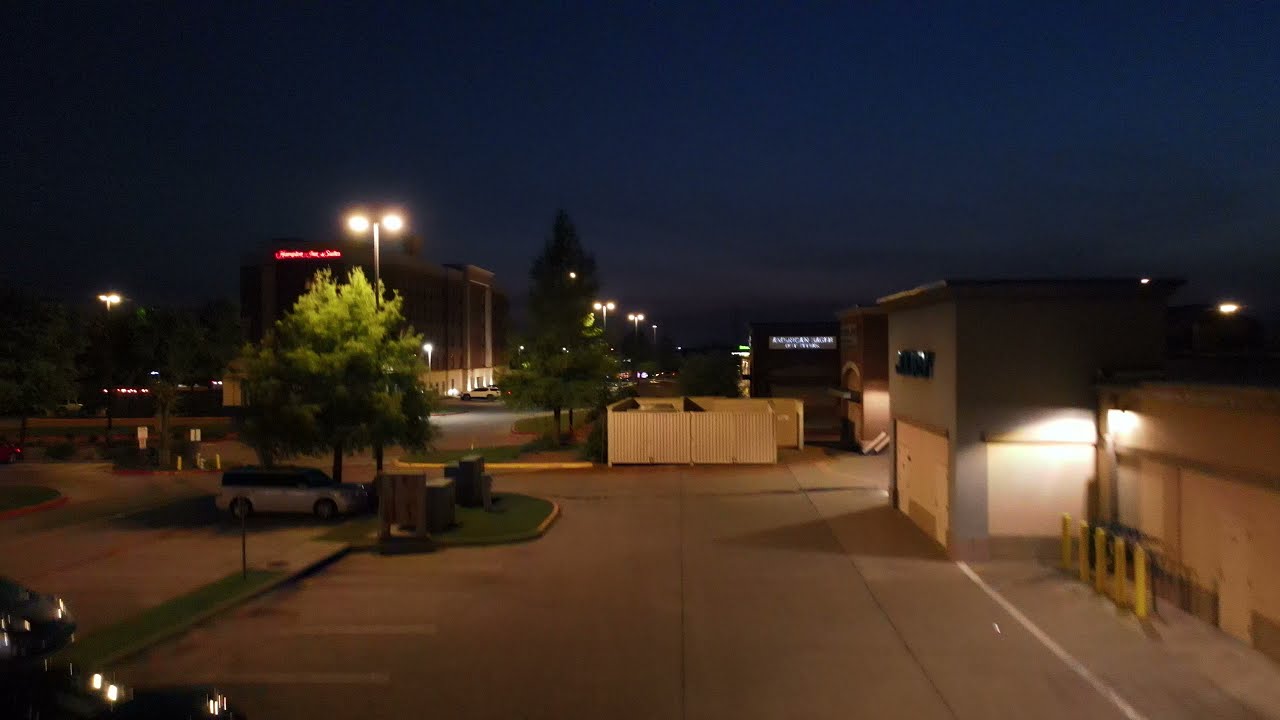This full-color nighttime photograph captures a horizontally rectangular parking lot scene, illuminated by numerous lights against a backdrop of dark blue and black skies. The parking lot itself is tannish brown and features a mix of buildings and vehicles. On the left-hand side, there is a medium-sized hotel, possibly a Hampton Inn, standing about four to six stories tall with a red, unreadable lit-up sign. Just in front of this hotel, and further left, are three parked cars, two near the lower left-hand corner and one directly beneath a tree in a grassy median.

Towards the right-hand side, the photograph shows the back side of some smaller brown buildings, including one with large closed doors likely used for receiving trucks. In the center of the scene, a tall white fence encloses trash bins, adjacent to a street lamp under which a white van is parked. Additional scattered vehicles can be seen faintly in the distance. The overall setting conveys a quiet, illuminated parking area in a small business district or hotel vicinity.